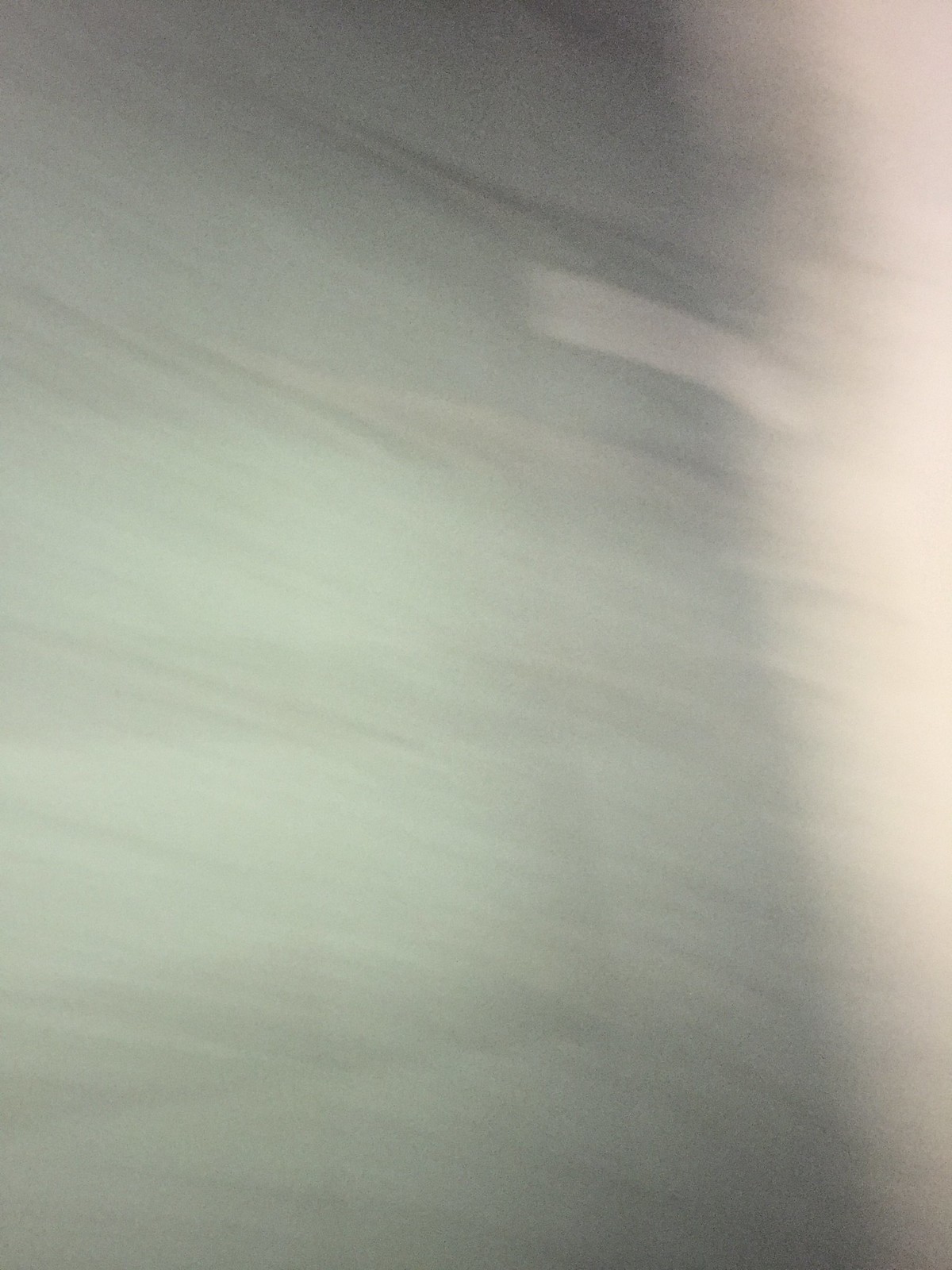The image presents an abstract, blurred background with an interplay of colors and shapes. Predominantly, a light green hue occupies much of the space, interspersed with dark shades of gray and black. Hazy, uneven lines cut across the scene, adding to the ambiguity. On the right side, an off-white color dominates, separated from the light green by a prominent diagonal black line. Near the top-right quadrant, there is a rectangular shape resembling masking tape, colored in off-white, lying across the intersection of the light green and off-white areas. The overall effect is a blend of abstract elements, creating a visual composition that invites interpretation.